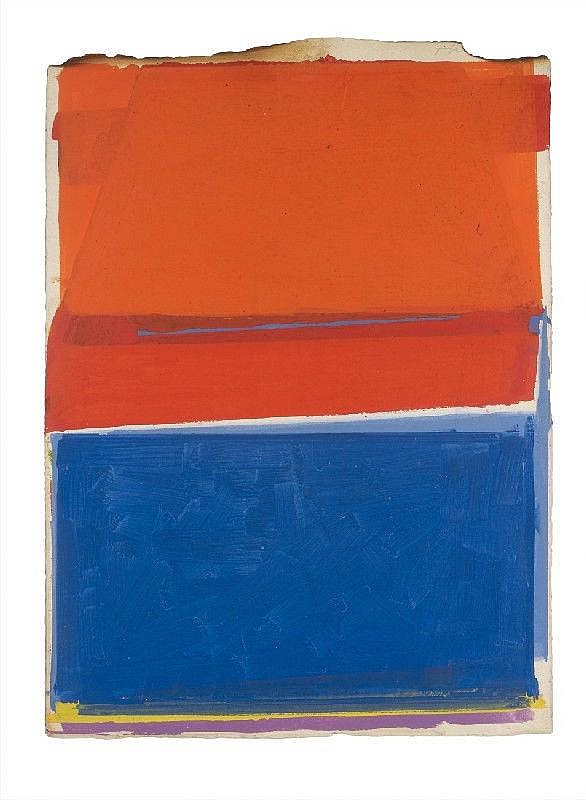The image depicts a long rectangular piece that resembles a Polaroid picture with irregular, torn, or possibly burnt edges, particularly at the top corners. The background of the image is a white or light beige canvas, with the torn sections revealing more of the white background beneath. The main content of the image is divided into two large, distinct rectangular sections. 

The upper section is an imperfect rectangular shape filled with a rich, burnt red or brownish-orange colored paint. The paint appears solid but reveals subtle brushstrokes along the top and sides. Approximately two-thirds of the way down the red section, a faint blue line spans across its width. 

A thin, angled white separation line divides the red and blue sections. The lower section is entirely painted in blue, with visible thick brushstrokes running in various directions. Below the blue section, a delicate strip of yellow and light purple lines extends across the entire width of the rectangle. The perimeter of the image retains the characteristic Polaroid picture border, maintaining the overall rectangular and bordered frame.